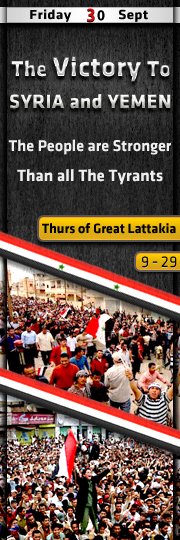The image is a vertically oriented graphic design combining text and photographs. At the top, a silver-gray strip with black text reads "Friday 30 Sept," where the number "3" in "30" is red. Below this, in white text on a black background, it declares "The victory to Syria and Yemen” and "The people are stronger than all the tyrants." Beneath these statements is a yellow bar with black text reading, "Thurs of Great Latakia," followed by another yellow bar indicating dates "9-29" in black text. Below these bars, there are horizontal stripes of red, white, and black, possibly representing the Syrian flag. 

The lower half of the image includes two photographs depicting large crowds, likely in protest. The first photograph shows a sea of people between buildings, stretching diagonally from the bottom left to the top right. Below another set of horizontal red, white, and black stripes, the second photograph focuses on a person standing amid the crowd, holding a flag matching the color scheme. This person stands slightly to the center-left, raising the flag triumphantly. Both images emphasize the theme of solidarity and resistance mentioned in the text above.